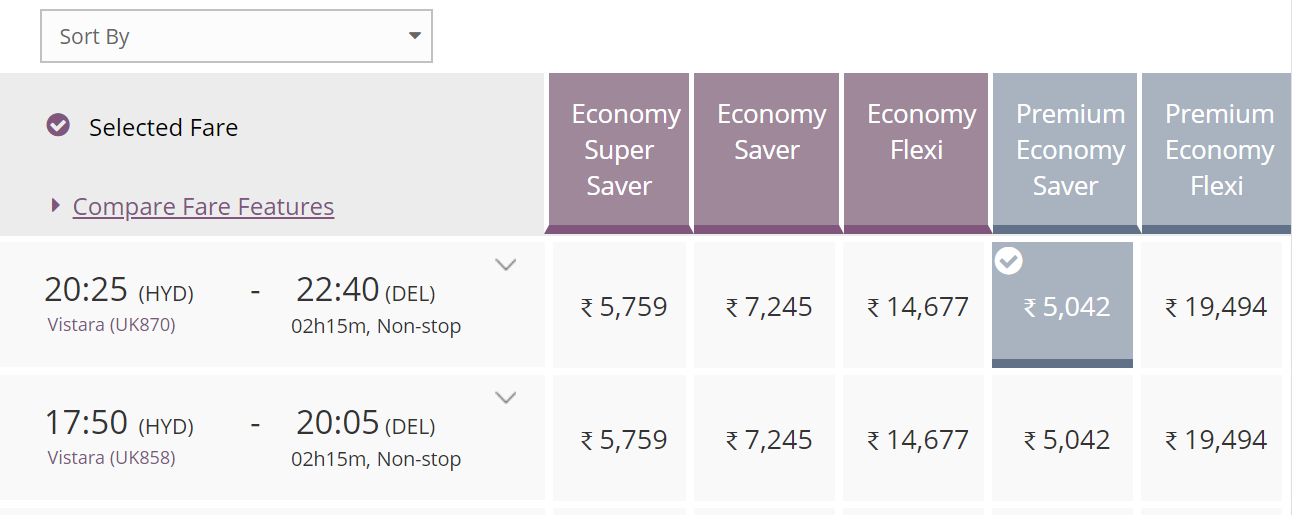The image depicts a screenshot from a travel booking website, which appears to be designed for booking flights, though it could possibly be used for buses or trains. The layout resembles a spreadsheet, with various columns and rows detailing different fare options. On the left side, the section is labeled "Selected Fare" with a link to compare fare features. Below this section, the selected trips are listed.

Currently, two trips are selected. The first trip is scheduled from Hyderabad (HYD) to Delhi (DEL), with a departure time of 20:25 and an arrival time of 22:40, indicating a non-stop flight duration of 135 minutes. The various fare options for this trip are displayed in five columns to the right: Economy Super Saver, Economy Saver, Economy Flexi, Premium Economy Saver, and Premium Economy Flexi. Each column lists the respective prices for the fare categories. 

The lowest fare, which is the Premium Economy Saver, is highlighted with a gray box and has been selected. The currency of the displayed prices is not specified in the image.